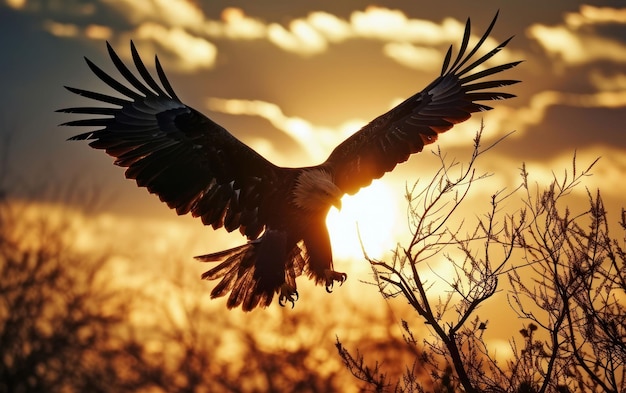In this horizontally aligned rectangular photograph, the main focus is a majestic bald eagle descending from the sky. The eagle's wings are spread out in a V-shape behind it, revealing the individual feathers. It features a distinctive white head and a small yellow beak, while its wings exhibit a dark brown or black hue. Its claws are fully extended, poised to land on or possibly seize prey from some bare tree branches situated in the lower right corner of the foreground.

The background of the image is a blur, emphasizing the eagle's detailed form. A field of brown stretches out indistinctly, suggesting blurred terrain or vegetation. The sky above is a mix of muted gray and brown tones, interspersed with white clouds. The orange-yellow glow of a setting sun, positioned slightly to the right of the eagle, adds a dramatic contrast and enhances the composition. The scene hints at either fall or winter, given the lack of leaves on the trees, and offers a serene yet powerful depiction of nature's raw beauty.